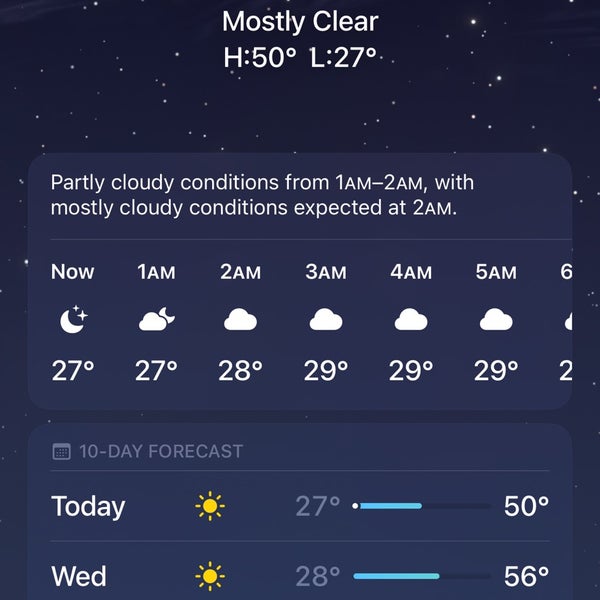The image appears to be a cropped screenshot from a smartphone displaying the weather forecast. The background features a dark, midnight blue hue with small dots simulating a star field, indicating a night sky. At the top center, "Mostly Clear" is written in white text, alongside the high (50°F) and low (27°F) temperatures for the day.

A dark blue rectangular section provides further details in white text, stating, "Partly cloudy conditions from 1 a.m. to 2 a.m. with mostly cloudy conditions expected at 2 a.m." Below this, an hourly forecast is presented in columns. The far-left column indicates "Now" with a crescent moon icon, representing clear skies, and a temperature of 27°F. Subsequent columns list the hours from 1 a.m. to 5 a.m., each accompanied by a cloud icon suggesting cloudy conditions. Temperatures for these hours progress as follows: 1 a.m. (27°F), 2 a.m. (28°F), 3 a.m. (29°F), 4 a.m. (29°F), and 5 a.m. (29°F). The far-right column shows the beginning of "6 a.m." but is cut off.

At the very bottom of the screenshot, a headline in light blue font reads "10-day forecast." Beneath this, only two days are visible: "Today" and "Wednesday." For "Today," a yellow sun icon with dots indicating sunshine is displayed, with temperatures 27°F (low) and 50°F (high). For "Wednesday," a similar sunshine icon is shown, with temperatures 27°F (low) and 56°F (high).